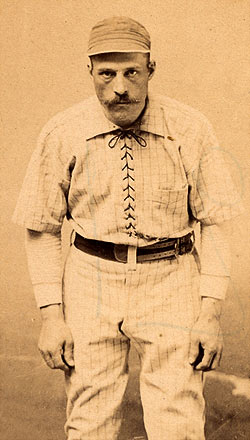This vintage photograph, with a brownish tint reminiscent of sepia, captures a baseball player from the late 19th or early 20th century. The monochromatic image prominently features the player in a central, standing position, looking directly into the camera with a focused expression. He is dressed in a classic, early baseball uniform that includes a striped white shirt with a high, laced front and white collar. Over his striped shirt, he wears a black leather belt, and the lower part of his uniform consists of matching white pinstriped trousers. His head is adorned with a billed baseball cap devoid of any logo, reflecting the styles worn in that era. The player, who appears to be Caucasian, sports a bushy handlebar mustache. He is standing on a grassy baseball field, with the background diffusing upward, adding to the timeless, historical feel of the photograph.